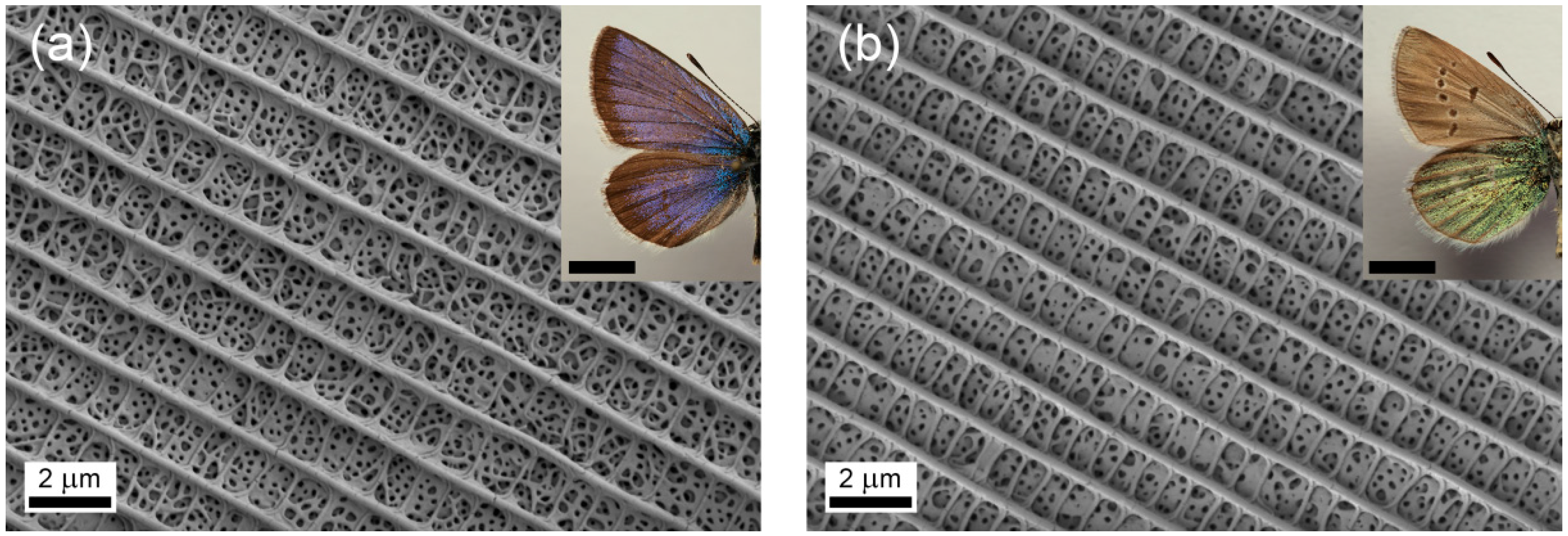This two-part horizontally rectangular image, segmented by a vertical white line, showcases both a photograph and an electron microscope view of butterfly wings. Each section is labeled in the upper left corner with "A" for the left image and "B" for the right image. The upper right corner of each section features a small photograph of a butterfly. Image A, on the left, displays a butterfly with a purple-bluish upper wing and a black body, with its wings shown in gray at a microscopic scale. Below this, a scale marked "2UM" helps gauge the level of magnification. The electron microscope view reveals rows of indented, web-like texture on the wing's surface. Image B on the right depicts a butterfly with a brown upper wing, a green lower wing, and a greenish body, typical of common insect coloration. The corresponding electron microscope view in B similarly zooms in on the wing’s texture, showing a variation in the microscopic structure that differs in color and pattern from A. Each half of this composite image combines to illustrate the intricate and varied microstructures present in butterfly wings.